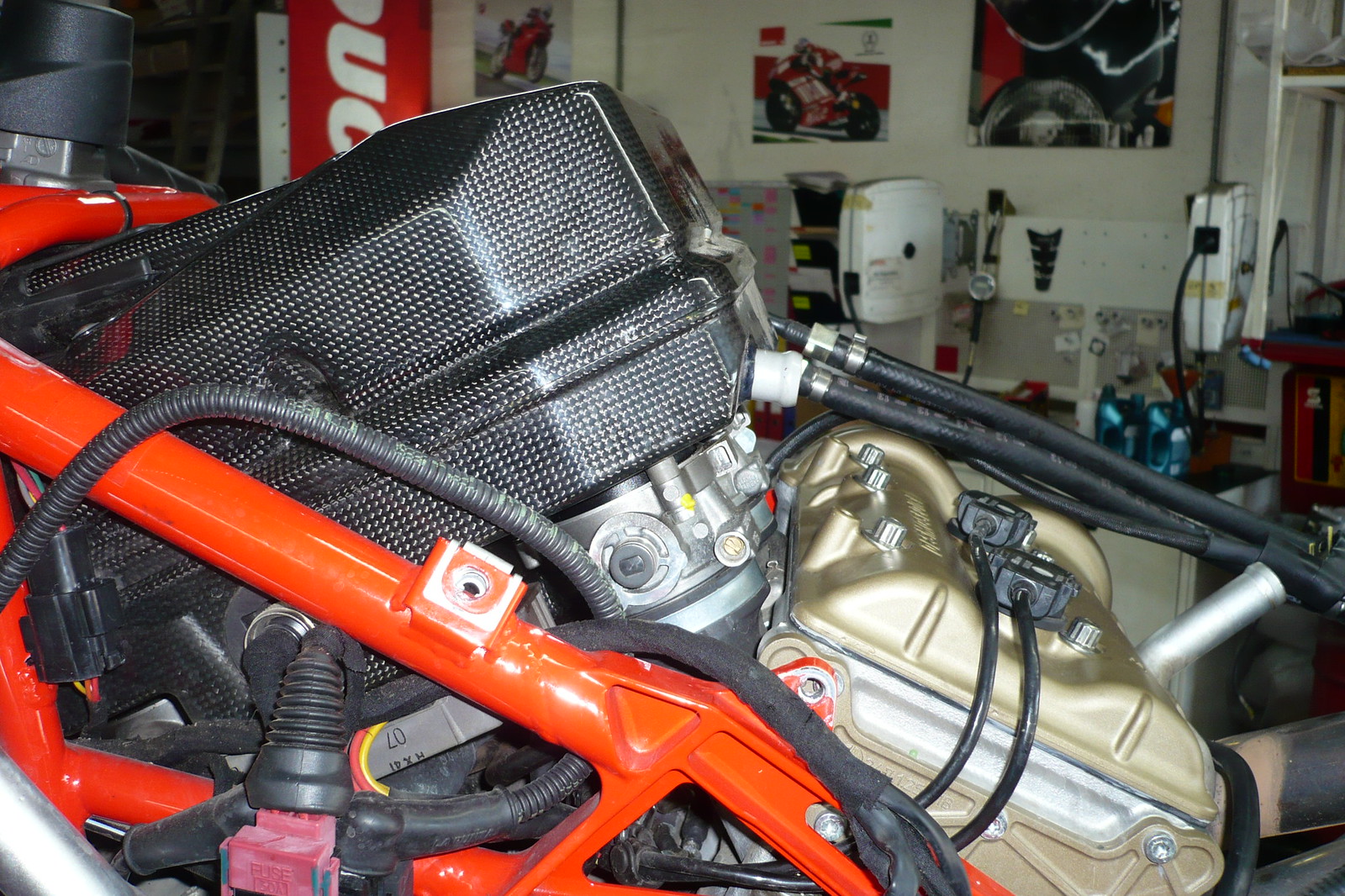In this detailed photograph taken indoors, we see a close-up of a meticulously clean, brand-new motorcycle engine set within a shop environment. The engine is prominently showcased in the foreground, featuring a sleek black top and a gold-painted metallic bottom, secured in a sturdy red-painted metal frame. The engine brims with detail, including black cords and wiring harnesses, silver terminals, and the marking "H41-07" clearly visible on one of the parts. 

To the mid-left of the engine, a red bar structure angles downwards, intersecting with additional red bars that frame the engine. In the background, a well-organized workshop setting unfolds: the wall is adorned with several vibrant posters of red motorcycles, suggesting the engine's ultimate purpose as a motorcycle component. The wall also features tool racks, a fabric bulletin board populated with numerous sticky notes, and a file holder. Additionally, bottles of oil and tools plugged into sockets add to the industrious ambiance. Among the posters, one prominently depicts a person riding a motorcycle, while another bears a sign that could be associated with "Dunlop" or "Ducati".